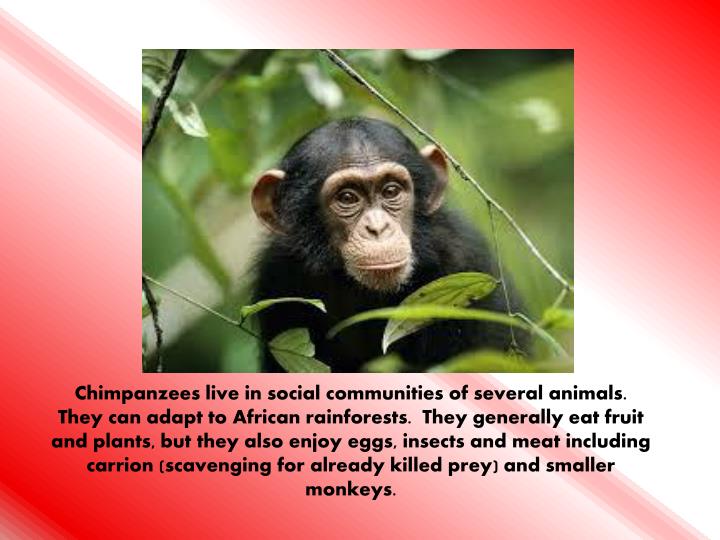The image features a small chimpanzee in a lush, green forest setting, surrounded by various branches and leaves. The chimpanzee, with dark black or possibly brown fur, dark brown eyes, and beige-colored ears, is situated amongst the foliage, with some branches near its head. The background highlights a striped red and white design with a diagonal white stripe running through the center. A caption beneath the image, written in black text, reads: “Chimpanzees live in social communities of several animals. They can adapt to African rainforests. They generally eat fruit and plants, but they also enjoy eggs, insects, and meat, including carrion, scavenging for already killed prey, and smaller monkeys.” The overall scene captures the essence of the chimpanzee's natural habitat, emphasizing its adaptability and social behavior.